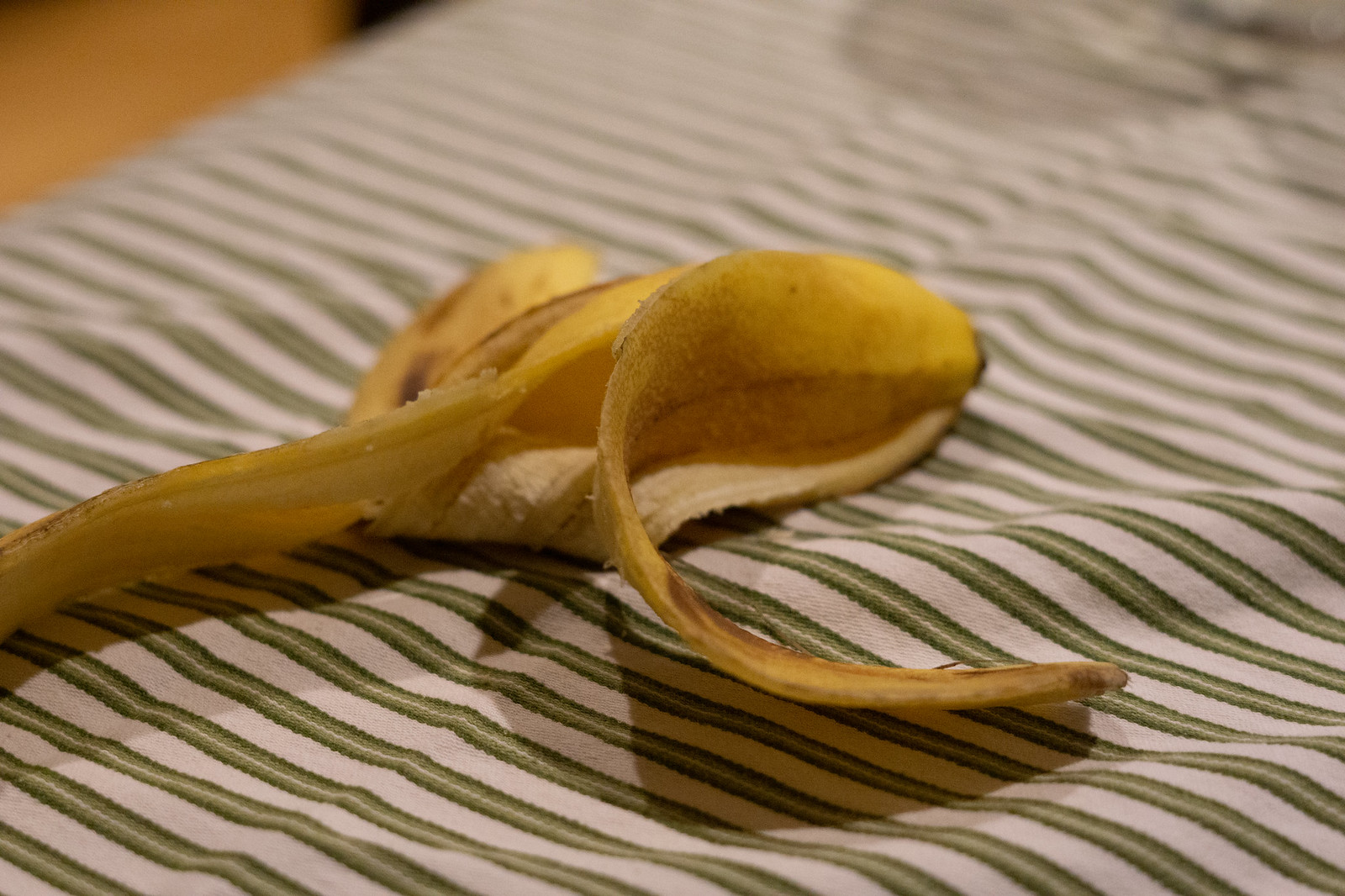The photograph showcases an empty banana peel artfully placed on a piece of white fabric with green pinstripes. The fabric, featuring horizontal stripes that are slightly diagonal from left to bottom right, includes tiny white lines down the center of the green stripes. The surface is not entirely flat, exhibiting slight undulations.

The yellow banana peel, accented with brown spots on its outer side and a whitish interior, is somewhat rolled up. Two sections of the peel extend towards the bottom of the image: one on the left side and the other forming a U-shape, bending towards the right. The light source is positioned at the top back, casting shadows underneath the banana peel and revealing an additional shadow from an obscure object at the back of the scene.

The focus of the photograph is intently on the front part of the banana peel, leaving the back of the peel and the fabric behind it slightly out of focus. This depth of field emphasizes the detailed texture and color of the closest sections of the banana peel.